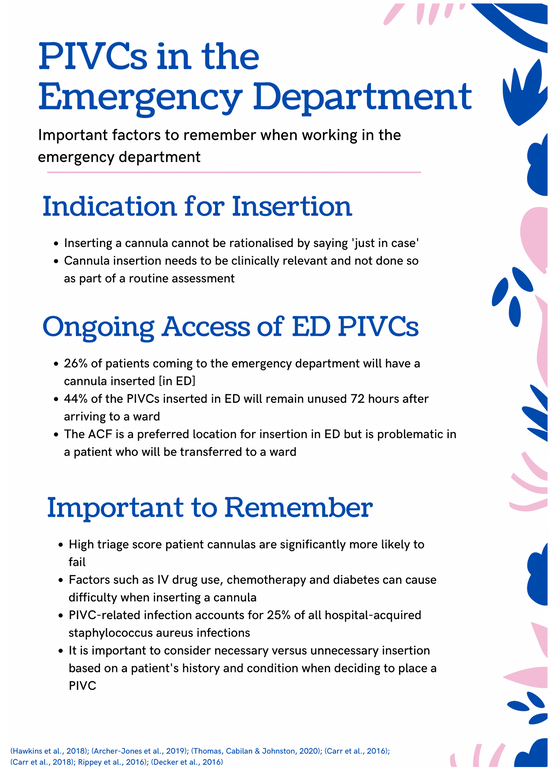This flyer, set against a white background with a pink and blue leafy design on the right side, is titled "PIVCs in the Emergency Department" in blue font at the top. Below, it outlines "Important Factors to Remember When Working in the Emergency Department," followed by "Indication for Insertion." Key points highlighted are that inserting a cannula cannot be rationalized by saying "just in case," and cannula insertion needs to be clinically relevant and not done as part of a routine assessment.

In the section "Ongoing Access of ED PIVCs," it states: 
- 26% of patients arriving at the emergency department will have a cannula inserted.
- 44% of PIVCs inserted in the emergency department remain unused 72 hours after arriving at a ward.
- The ACF, while a preferred insertion site in the emergency department, is problematic for patients who will be transferred to a ward.

Finally, under "Important to Remember," the flyer includes the following points:
- High triage score patients’ cannulas are significantly more likely to fail.
- Factors such as IV drug use, chemotherapy, and diabetes can cause difficulty when inserting a cannula.
- PIVC-related infections account for 25% of all hospital-acquired Staphylococcus aureus infections.
- It is crucial to consider the necessity versus unnecessary insertion based on a patient's history and condition. The source of the information is attributed to Thomas Cabellan and Johnston 2020.